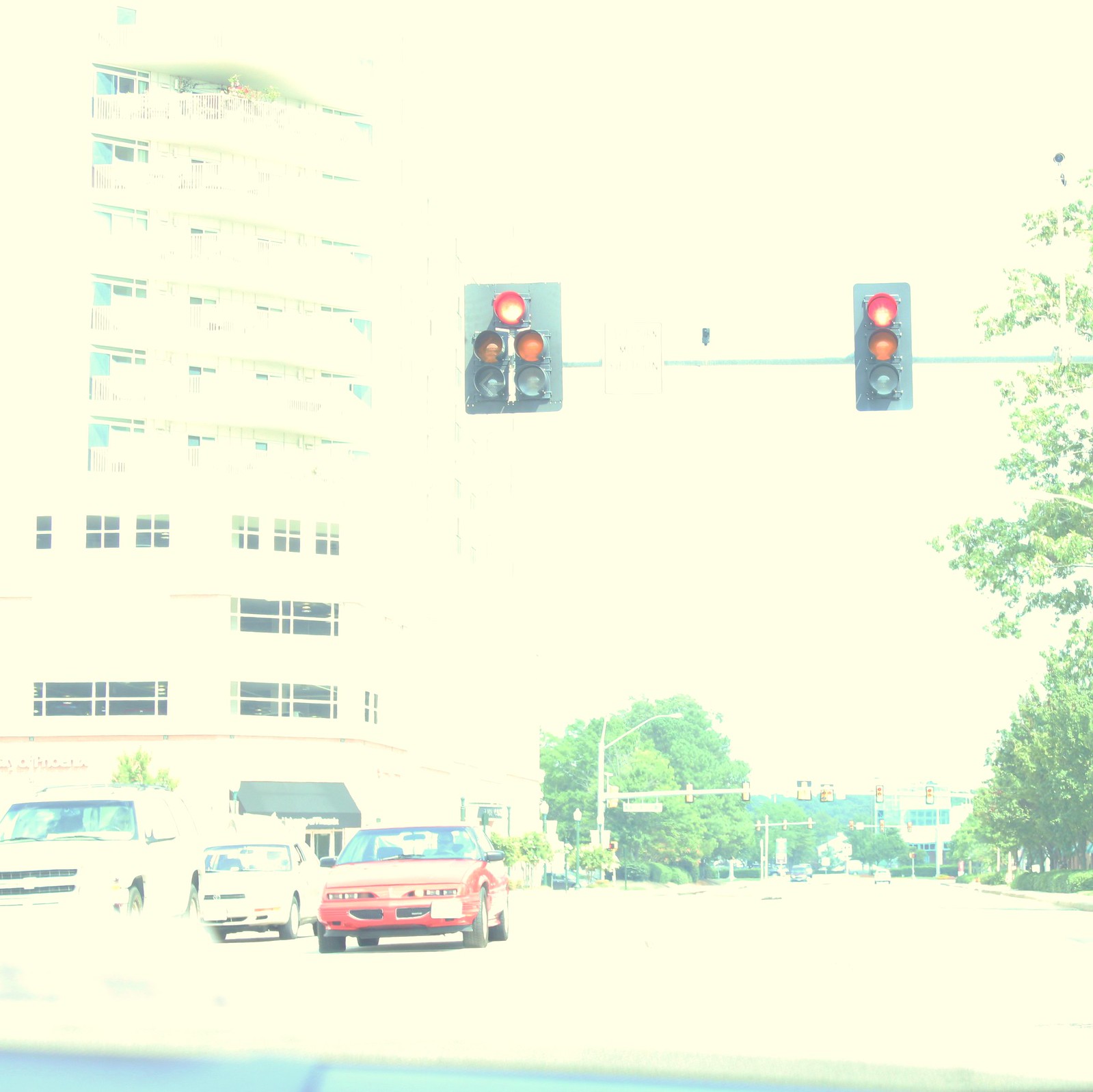The image presents a driver's perspective from within a vehicle, capturing a brightly lit scene. The intense white light pervasive in the picture renders almost everything a predominant white hue. At the very bottom of the image, there is a faint light blue strip that likely represents the dashboard of the vehicle. The road ahead is also illuminated to appear almost entirely white. 

To the left, two cars are visible; one is entirely whitened out by the light, while the other distinctly appears red. These cars are viewed from the front, indicating they are part of the opposite flow of traffic. In the distance, a traffic light is present but faded to the extent that its color is indiscernible. 

There is a green sign that stands out in the background, and to the left, a towering, multi-story building with black windows is prominent. Adjacent to this building, a green tree stands out, followed by another cluster of green leaves further to the right. Dominating the upper portion of the image, the sky shines an almost unnaturally bright white, contributing to the overall high-exposure or potentially overexposed appearance of the scene.